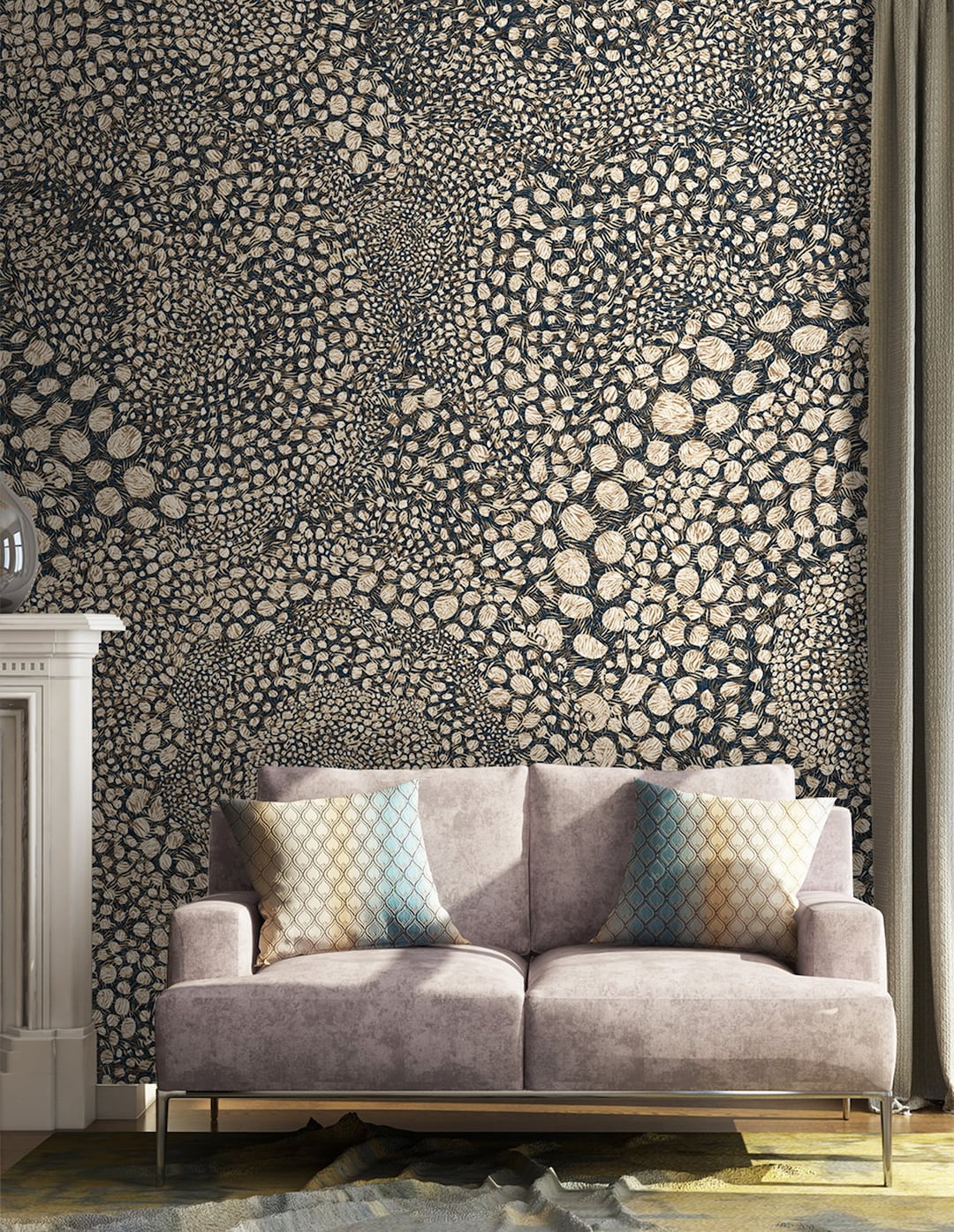This photograph captures a cozy indoor living area with a meticulously detailed backdrop. The wall features an intricate, artful wallpaper with a dark navy blue to almost black background, adorned with swirling circular patterns in varying sizes, resembling seashells or the overlapping inside of blood cells. These patterns, in shades of white and gold, add depth and texture to the space. In front of this ornate wall stands a plush, light lavender suede love seat with metallic feet, accompanied by two throw pillows in a diamond pattern of white, turquoise, and yellow. To the left of the love seat, the image includes a glimpse of a white mantel adorned with gold details, connected to a partial view of a fireplace. The floor hosts a slightly wrinkled gray and tan carpet, completing the warm, inviting ambiance of the room.